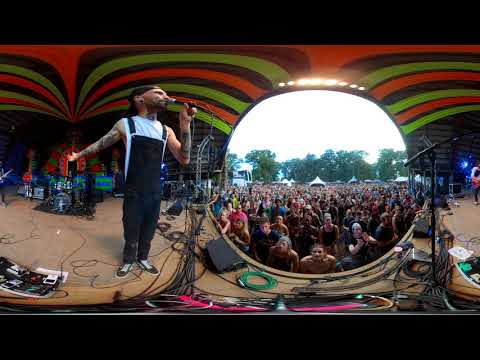A man in dark overalls and a white t-shirt, adorned with tattoos, stands on a brown stage, holding a microphone. The stage is set up with a drum set, guitar pedals, and various sound equipment, with numerous black wires running across it. The stage is covered by a canopy featuring an interesting striped pattern in orange, brown, green, and black. The scene is captured in a distorted, fish-eyed panoramic view, centering a crowd of concert-goers who appear in a warped circular formation. Behind the crowd are tall trees under a bright white sky, and some white tents are visible amidst the audience. The overall distorted image gives the impression of the performer and crowd being slightly misshapen, with the performer appearing smaller and with a disproportionately large head.